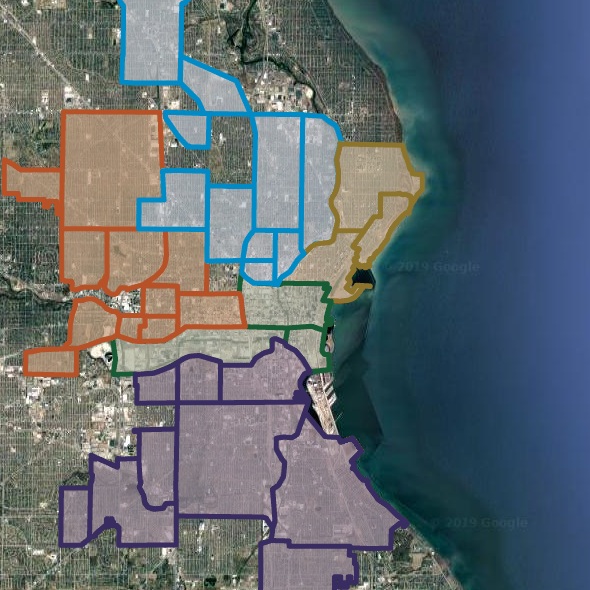The image is a detailed satellite view from 2019 Google Maps, featuring a coastline that runs from midway across the top, curves toward the right, and ends near the bottom right corner. On the right side, there is a body of water, which might be part of a river or tributary system cutting into the landmass. The lighter blue font on the water reads "2019 Google." The left side showcases a landmass, broken into grid-like patterns, with certain regions outlined and color-coded in turquoise, orange, dark gold-yellow, green, and dark violet-purple, which may represent various districts or zones. Not all areas are covered by these color-coded grids; some areas display just the streets and roadways with visible blocks. Additionally, there appears to be part of a dock or harbor that’s not encompassed by the color-coded zones. The superimposed colorful outlines add vibrancy to the otherwise muted satellite representation.